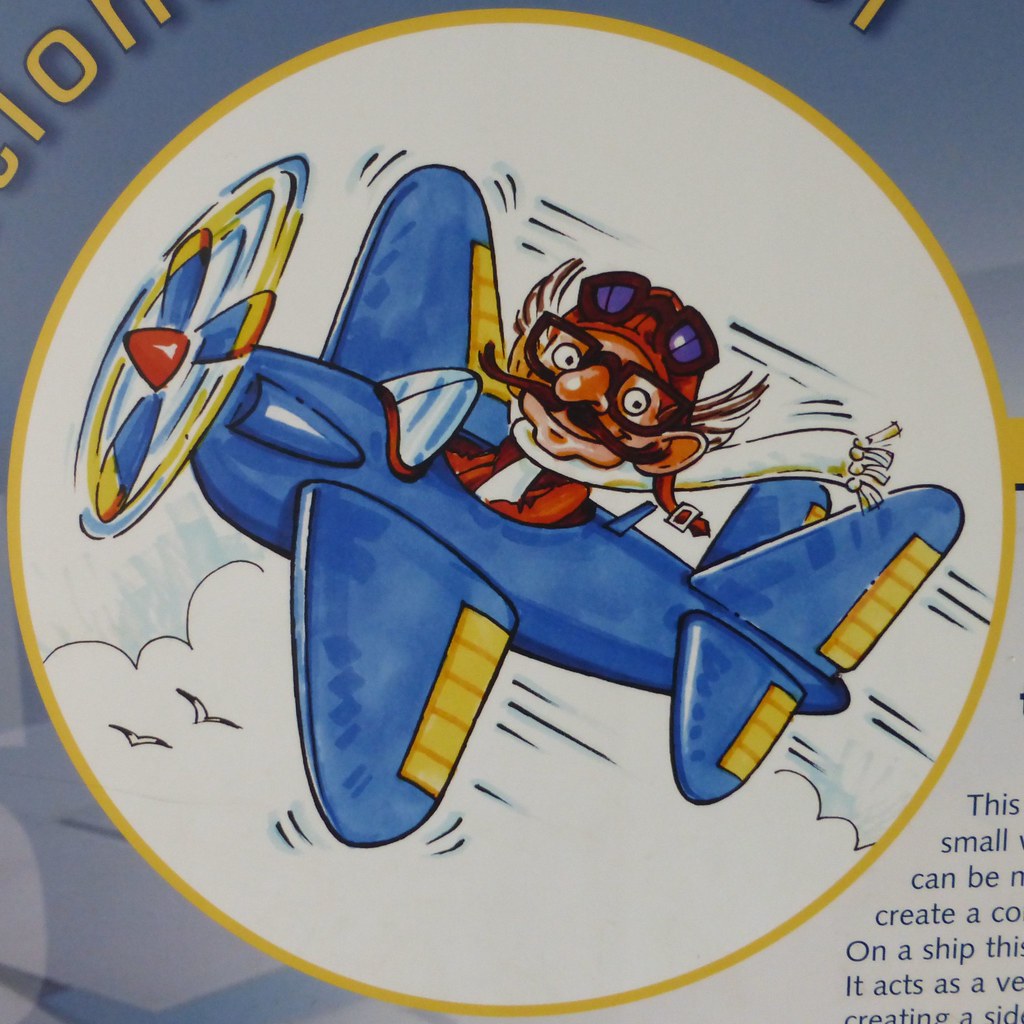The image is a detailed illustration featuring a cartoon man piloting a small, blue airplane amidst floating clouds. The man, depicted with brown glasses and a long brown mustache, wears a red hat adorned with brown goggles. His attire includes a red jacket and a long white scarf that blows behind him in the wind. The airplane, primarily blue, has yellow accents on its wings and tail and displays some ocean lines. The scene is encapsulated within a yellow round frame, with the top, bottom, top two corners, and bottom right-hand corner of the image slightly cropped. Additionally, the propeller is illustrated to give the impression of spinning, adding to the dynamic feel of the illustration. In the bottom right corner, there is some partially visible text in yellow and dark blue fonts, although it's mostly cut off. The image appears to be a close-up photo of a poster, leaflet, or even a collectible plate, potentially created using watercolor techniques.